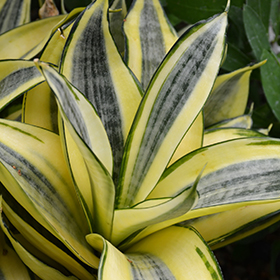This detailed close-up image showcases a vibrant plant filling the entire square frame. The plant features long, pointed leaves that radiate from a central core, resembling a snake plant. Each leaf is intricately patterned, with a gold outer band and a predominantly green edge. The central portion of the leaf is gray, adorned with two darker stripes running through it, creating a striking contrast against the yellow midsection. The leaves vary in width, with some being broader and almost teardrop-shaped, giving the plant a dense, layered appearance. The background reveals additional green leaves, yet there's no visible stem or flowers, drawing all attention to the intricate foliage arrangement. This tropical-esque plant brings to mind the look of layered banana peels due to the unique coloration and striping, adding to its captivating visual appeal.